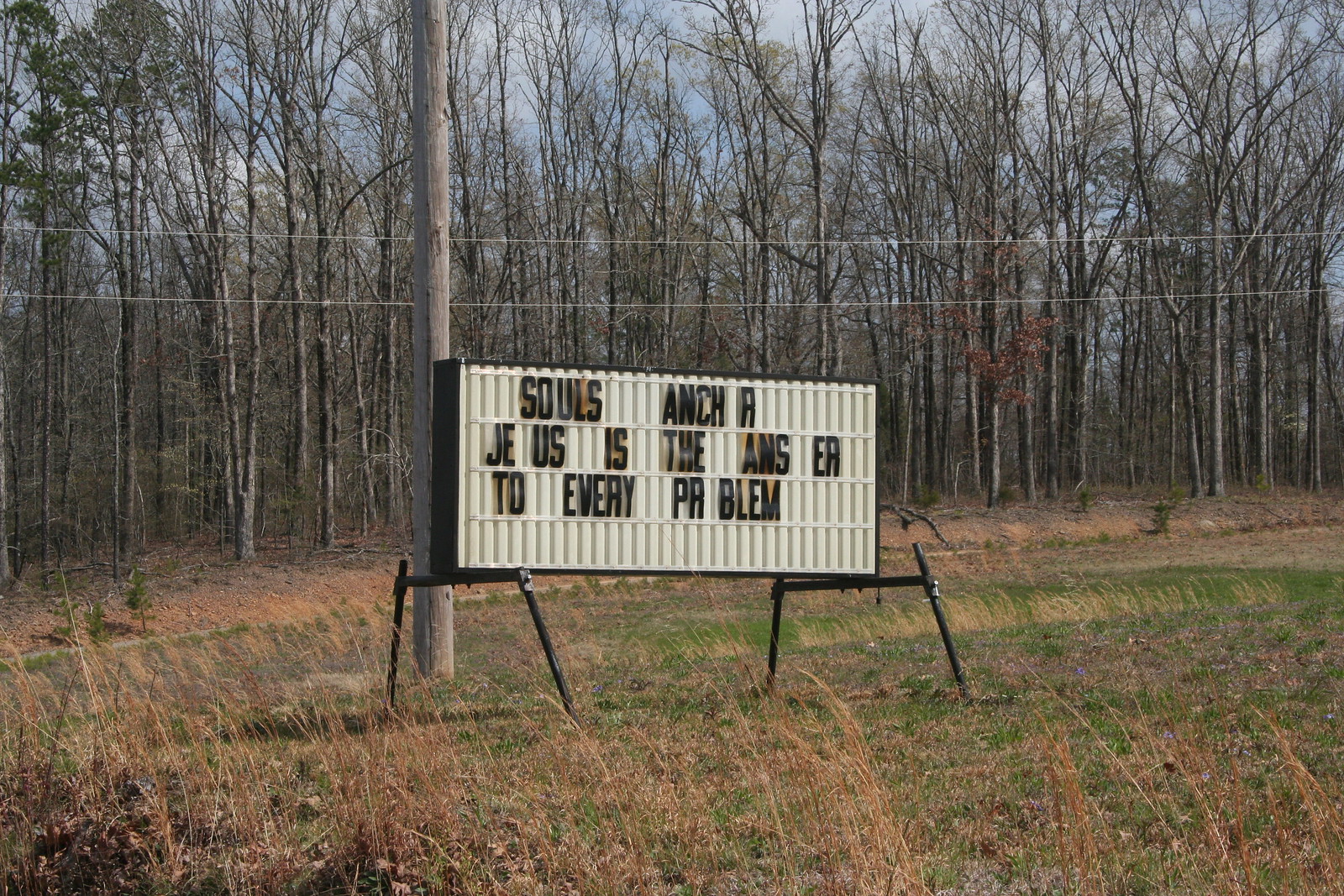The image captures a horizontal outdoor scene likely taken along a rural roadway. Centered in the frame is an old, white portable sign with a black metal frame, leaning against a telephone pole strung with power lines. The sign, showing its age and wear, is situated on a barren and slightly grassy hillside. The short green grass in front gives way to longer, golden, hay-like grasses. Behind the sign and pole, a sparsely-leaved, brownish forest stretches under a cloudy blue sky, suggesting a fall setting. The portable sign, meant for slotting in individual letters to create messages, displays an incomplete religious message. It reads: "souls A-N-C-H-R Jesus is the ans-er to every pr-blem," with several letters missing such as the first 'O' in "anchor," the first 'S' in "Jesus," the 'W' in "answer," and the 'O' in "problem." The desolate setting and wear on the sign emphasize the passage of time and the persistence of the message despite its imperfections.